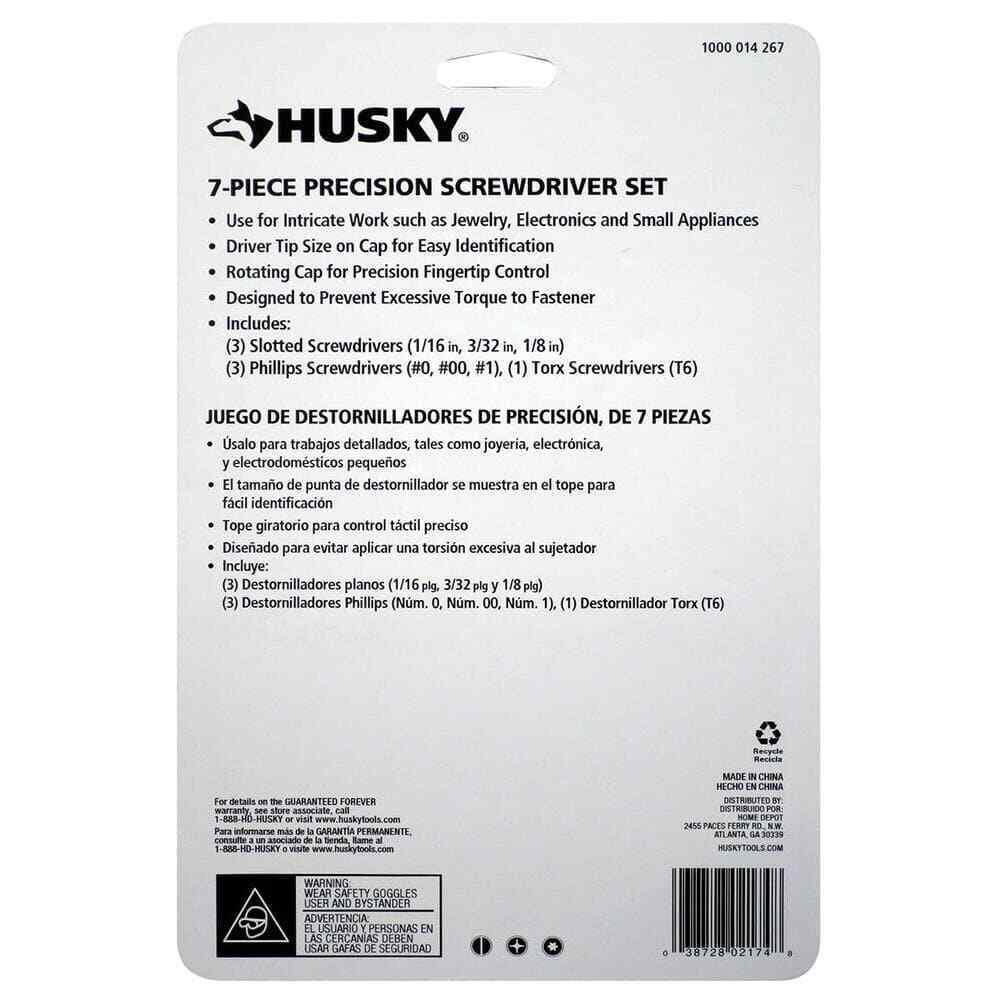The back of the package for a Husky brand 7-piece precision screwdriver set prominently features the Husky logo, including a dog's sideways profile, all in black and white. At the top left, "HUSKY" is displayed in all caps. The package is designed to hang on a metal hook in a store, evident by the cutout in the center. Below the logo, the text details the screwdriver set's uses, ideal for intricate work such as jewelry, electronics, and small appliances. The set includes three slotted screwdrivers (1/16", 3/32", and 1/8"), three Phillips screwdrivers (#0, #00, and #1), and a Torx T6 screwdriver, with the driver tip sizes indicated on the caps for easy identification. Additional features mentioned are the rotating cap for precision fingertip control and a design that prevents excessive torque to fasteners. This information, along with general safety warnings, a barcode, recycling information, and a "Made in China / Hecho en China" label, is repeated below in Spanish.